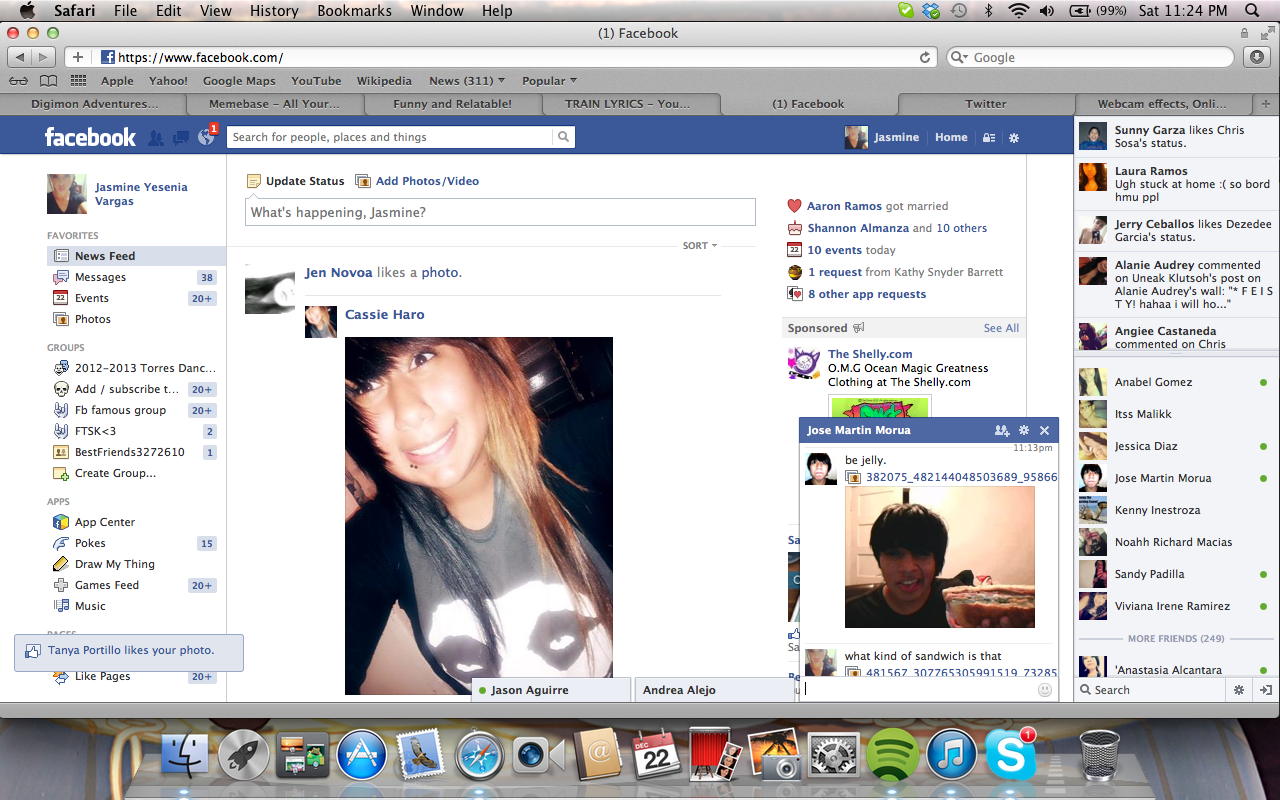The image is a detailed screenshot taken from a MacBook, showing the Facebook profile of Jeannine Vargas, though other names like Yasmin Yesenia Vargas and Jasmine Yacina Vergis are mentioned. The upper tab displays typical Mac indicators including the Apple logo and menu options for Safari such as File, Edit, View, History, Bookmarks, Window, and Help. It's Saturday at 11:24 PM, with the battery life at 99%. 

On the Facebook webpage (www.facebook.com), the profile of Jeannine Vargas is visible with standard elements like the news feed, messages, events, and various buttons. The profile includes a recent post by Cassie O'Hara, featuring Cassie wearing a black t-shirt with a white image that appears to be a person's face with darkened eye makeup. There's an ongoing text conversation visible with Jose Martin Maria, albeit difficult to read due to the small font size. The bottom of the desktop displays several application icons including Safari, Spotify, Apple Music, Skype, the Trashcan logo, and the Calendar. Additionally, there are several other browser tabs open.